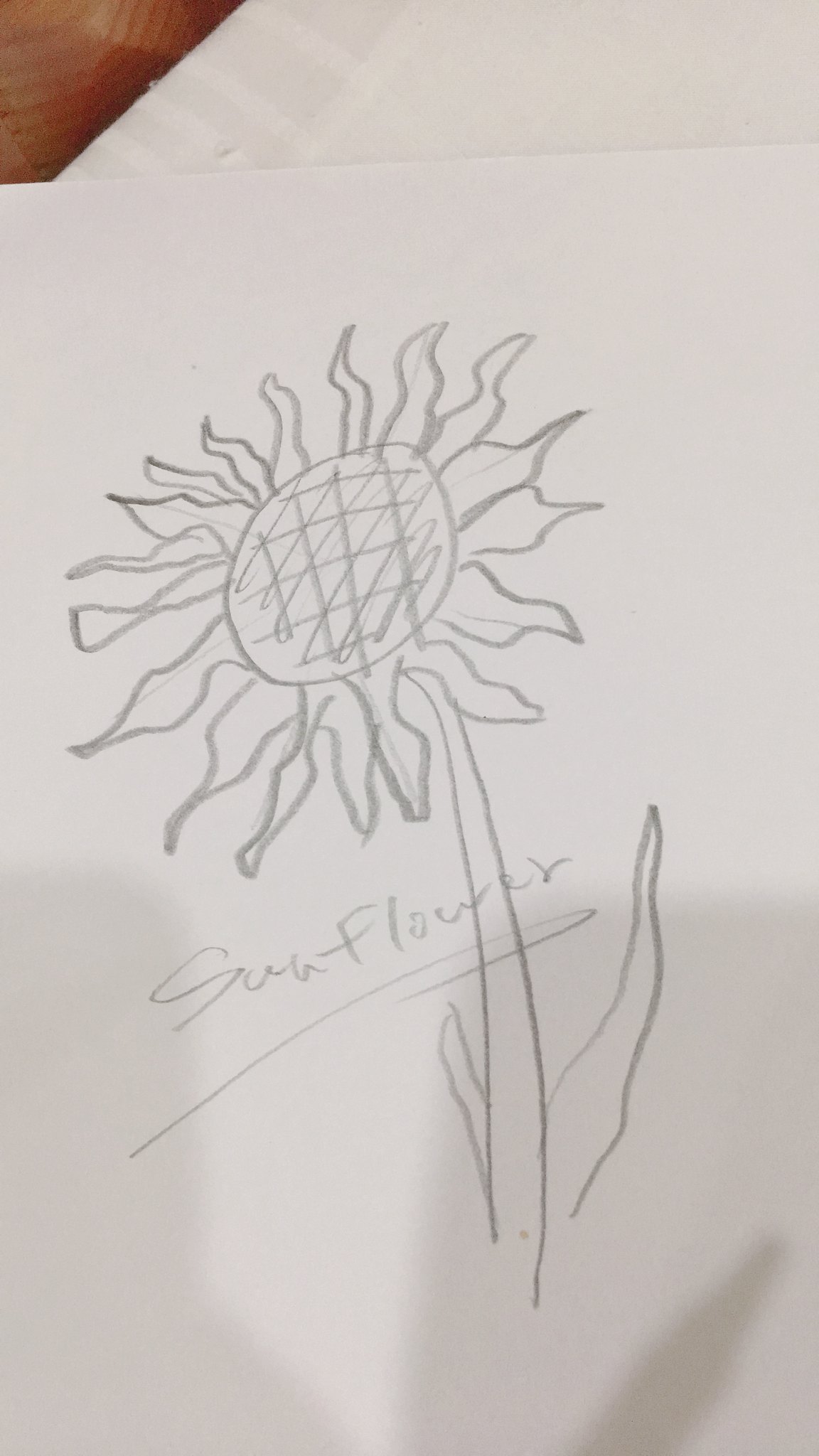This image captures a simple yet charming pencil drawing of a sunflower on a white piece of paper. The drawing features two clean lines for the stem, accompanied by two elongated leaves positioned near the base. Atop the stem blooms the unmistakable sunflower, characterized by a large, shaded oval center, surrounded by approximately 20 petals emanating outward in a flame-like shape, giving it that classic sunflower appearance. The word "sunflower" is scrawled across the middle of the drawing, the letters extending across and slightly above the stem, underlined for emphasis. The photograph of this sketch appears to be situated on white fabric, with a hint of a brown wooden background visible in the upper left corner, suggesting the paper is resting on a table. Overall, it presents a straightforward, endearing visual created perhaps by a young artist or someone with modest drawing skills.